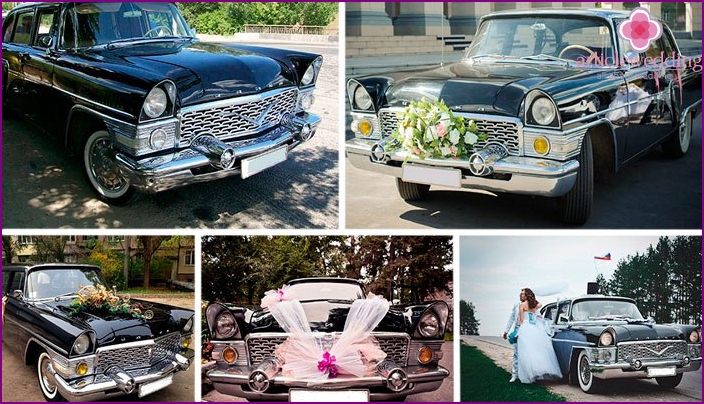The image is a collage of five outdoor photographs featuring a shiny black vintage car from the 1950s adorned with chrome and wedding decorations. The photos primarily showcase the car with various floral arrangements, including pink and white flowers and a prominent pink ribbon on the front grille.

In the upper section of the collage, two large photos highlight different angles of the car. One photo displays a logo, partially readable, indicating something related to a wedding photography service. 

The bottom section comprises three smaller photos. The bottom middle one presents a front view of the car with trees in the background, while the bottom right features a newlywed couple standing beside the car against a backdrop of green trees, a cloudy sky, and a lush lawn. The left bottom photo offers a side view of the car parked in a light-colored neighborhood, surrounded by houses, trees, and a railing.

The entire collage emphasizes the festive and celebratory atmosphere of a wedding, with each photo capturing different details and perspectives of the elegantly decorated car.